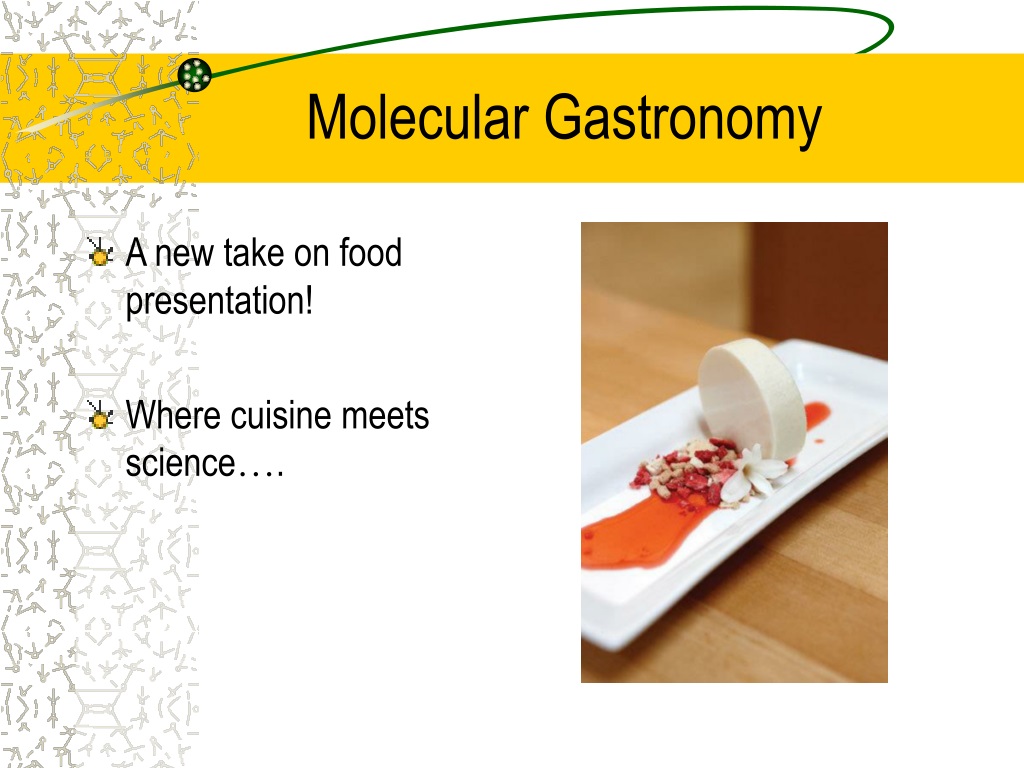The image depicts the front page of a PowerPoint presentation titled "Molecular Gastronomy." The title, written in black text, is placed within a thick yellow horizontal bar at the top of the slide. Overlaying the yellow bar is a circular green line enclosing a green ball with white specks. On the left side of the slide, there's a grayish-green vertical band featuring pencil sketch-like symbols, possibly representing molecular notations. Below this, there are two yellow bullet points: the first one states "A new take on food presentation," and the second reads "Where cuisine meets science." To the right side of the slide, there's a detailed photo of a plated dish: a white, circular food object, adorned with red sauce on each side, and garnished with what appear to be mixed red and white nuts or berries, presented on a rectangular porcelain plate.